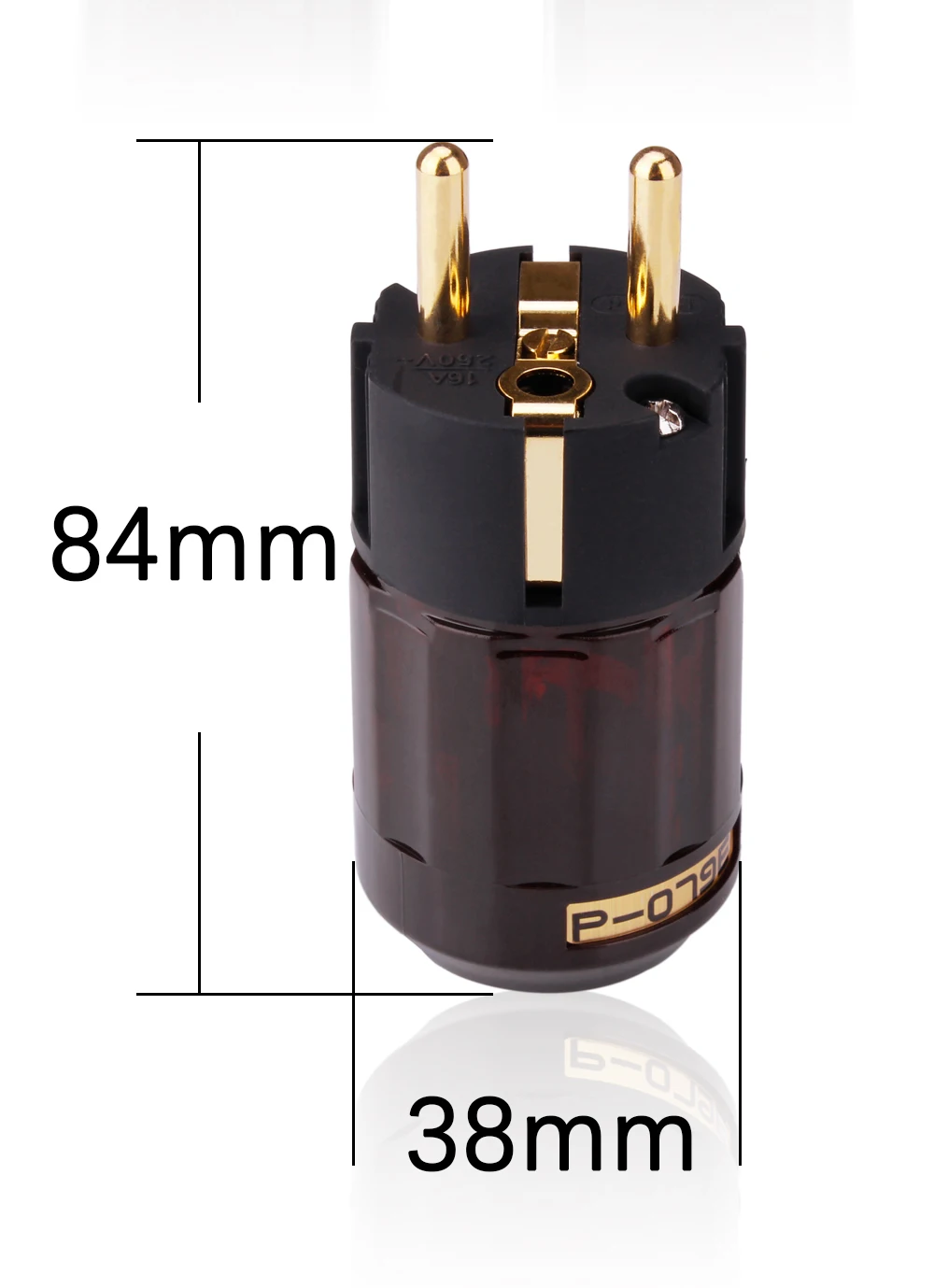This is a close-up image of a cylindrical plug designed for a different country, set against a white background. The plug, standing upright with its base down, features two rounded, gold-colored prongs at the top. The main body of the plug is predominantly black, occupying about 40% of its height, and it transitions to a semi-transparent, brown-colored plastic lower section. A gold connector extends down from the recessed area on the black section along the plug's side. The plug also features a gold label near its bottom, marked with "P-079" in black text, though the full text extends off-screen. Detailed measurements are annotated on the image: the height of the plug is labeled as 84 millimeters on the left side, and its width is marked as 38 millimeters with lines extending from the left and right sides. The plug is casting a shadow along its base, emphasizing its three-dimensional form.